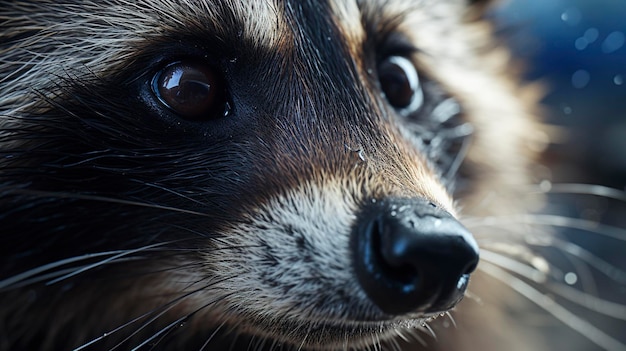The image features a close-up, color photograph of an alert raccoon, showing a detailed three-quarter view of its head and face. The raccoon's large, shiny black nose is prominent against its whitish muzzle, and its wide, open eyes add to its eager or surprised expression. Signature features like the black band stretching across its eyes and nose, as well as the streak of white fur above its eyes and head, are easily visible. Numerous whiskers shoot out from its snout and cheeks. The raccoon is turned slightly to the right, with its closed mouth enhancing a sense of readiness. The backdrop presents a blue hue with an unclear falling substance, possibly water, adding a dynamic element to the scene. The lighting suggests the photo might have been taken outside at night, with some light illuminating the raccoon's face against the darker background.